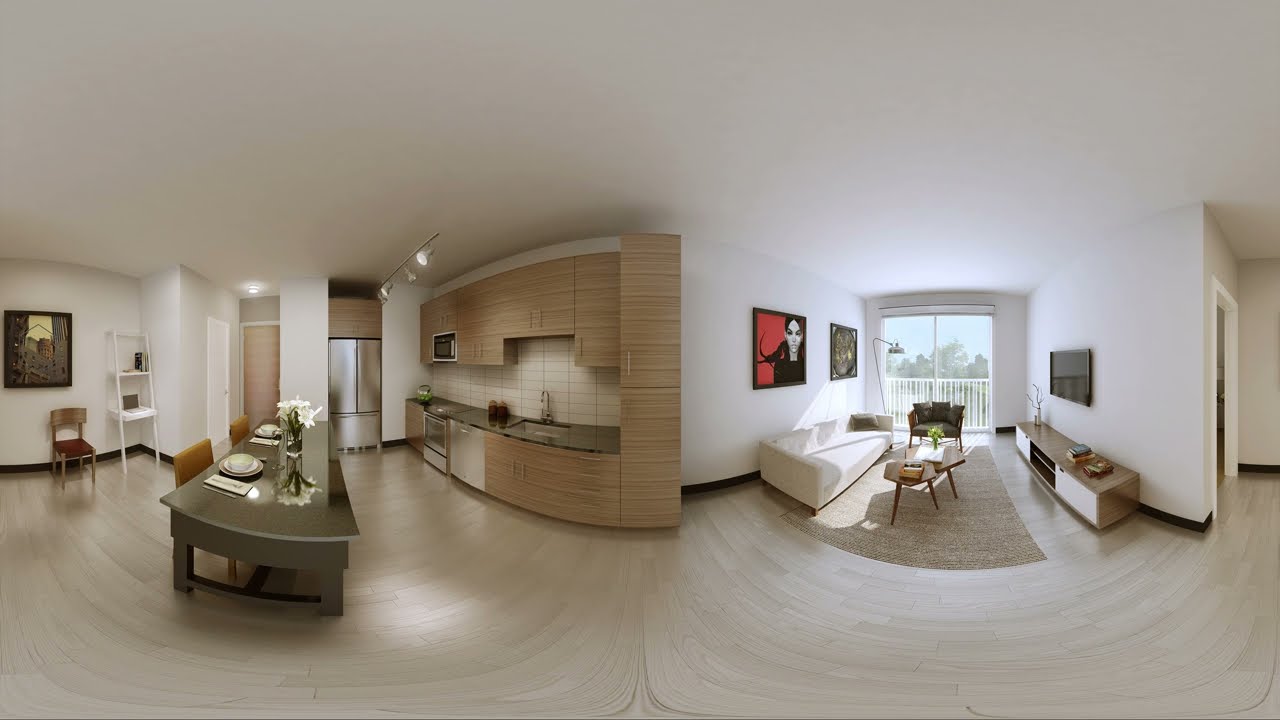The image depicts a daytime interior setting of an apartment captured in a horizontally aligned rectangular picture. The scene is comprised of two main areas divided into the kitchen on the right and the living room on the left. 

The kitchen features brown hanging cabinets and matching brown lower cabinets that extend from the countertop to the ground. The black countertop houses a sink, a stove, an oven, and a washing machine positioned centrally. To the left of the kitchen area, there is a dining space with a gray table and brown cushioned chairs. The table is set with dinner plates, silverware, and a vase with flowers.

On the left side of the image, the living room is furnished with a white couch against a white wall adorned with two pictures above it. There is a black TV mounted on this wall, and in front of the couch are a couple of small tables positioned on a rug. The far end of the living room features a sliding door leading to a balcony, which is lined with a white railing and overlooks a view of trees.

The apartment has a white ceiling and tiled flooring with a swirled pattern of white and light brown or beige. The image is detailed with a variety of colors including white, black, brown, gray, tan, and subtle hints of red and green, suggestive of the indoor setting being well-lit, possibly during the middle of the day. The overall composition of the photograph captures a cozy and organized space with a blend of modern and comfortable furnishings.